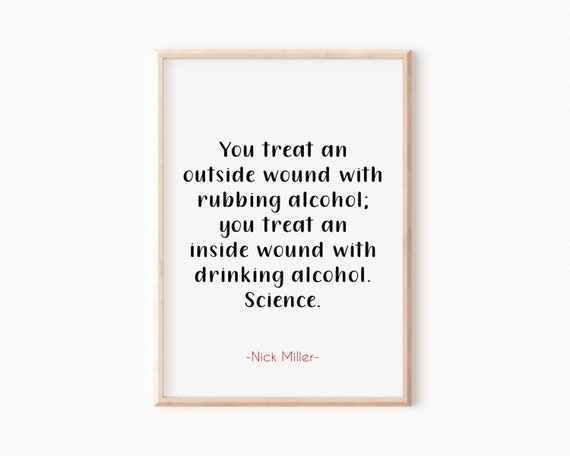The image portrays a piece of text against a plain white background, framed by a beige-colored wooden frame that casts a light gray shadow to the right. Inside the pink frame, the text humorously reads, "You treat an outside wound with rubbing alcohol. You treat an inside wound with drinking alcohol. Science." The main quote is displayed in a larger, black comedic-style font, while the author's name, "Nick Miller," appears in a smaller pink font below, enclosed by pink dashes. The overall design is minimalistic, with ample white space surrounding the text.